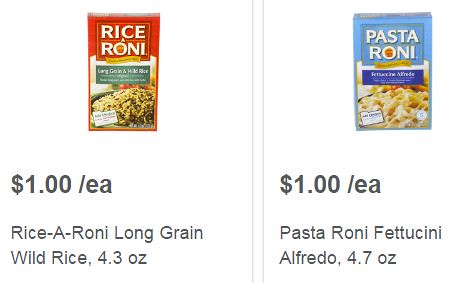The left image displays a red package of Rice-A-Roni Long Grain & Wild Rice, prominently featuring the iconic Rice-A-Roni logo in bold white letters at the top. The packaging includes an appetizing photograph of a plate heaped with light and dark brown grains of wild rice, presumably showcasing the product when prepared. 

The right image illustrates a box of Pasta-Roni Fettuccine Alfredo. The box is light blue and also displays the recognizable Pasta-Roni logo at the top. An enticing photograph of rich, creamy fettuccine noodles covered in a classic white Alfredo sauce is featured on the front, suggesting a delicious, ready-to-prepare meal.

Both items are listed with a clear price of $1 each, indicating their affordability on what appears to be an online grocery store ordering app.